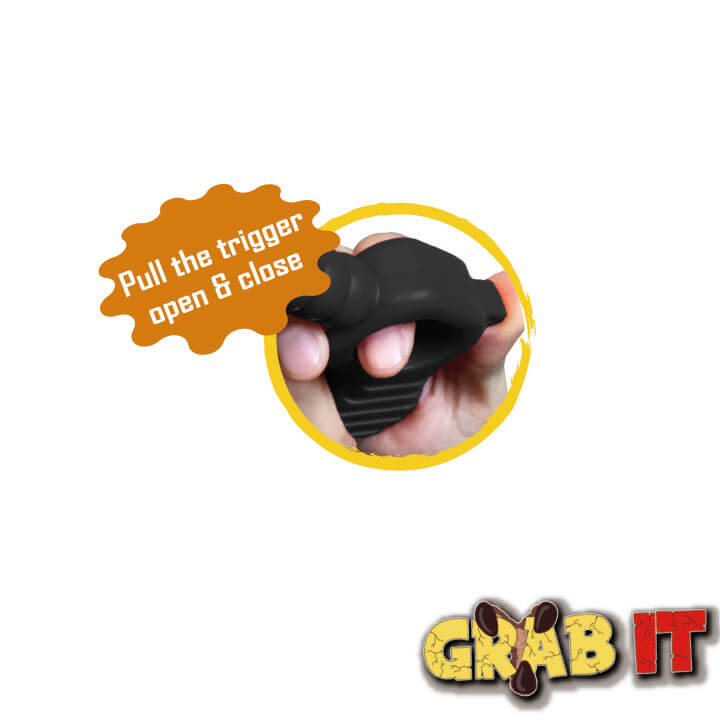The image features a minimalist white background devoid of borders, with bold text and intriguing graphics that suggest an advertisement for a product named "GrabIt." At the bottom of the image, the bold text "Grab It" appears, with "Grab" in yellow and "It" in red, both words exhibiting crack-like details. A brown claw, with its tips darker in hue, emerges from behind and appears to grasp the letters "R" and "A." Shadowed gray outlines enhance the text, giving it a three-dimensional effect.

Above this text is a circular image showing a hand gripping a black object, with fingers visible through a trigger-like hole, suggesting some sort of hand-operated device. Adjacent to this image, an orange oval bubble, reminiscent of a playful Nickelodeon aesthetic, contains the command "pull the trigger, open and close" in white text, hinting at the operational mechanism of the product. The composition and visual elements clearly aim to draw attention and generate curiosity about the functionality of "GrabIt."